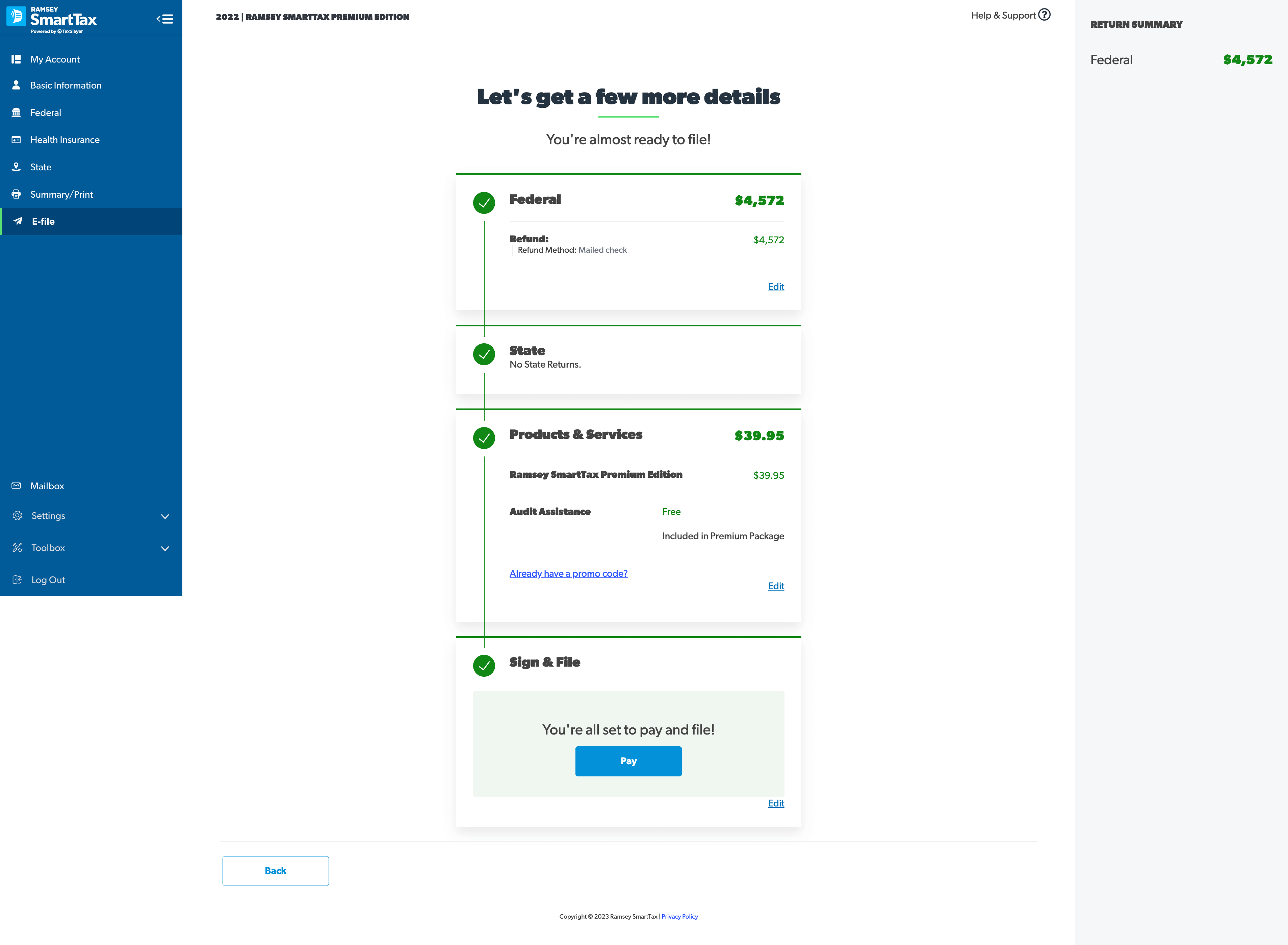The image features a user interface on a white background. On the left side, there's a blue sidebar with a small light blue box containing white text that reads "Smart Tags." The sidebar also includes a left arrow, three horizontal lines, "My Account," and an "Edit" option highlighted in blue. Below these, there are several other options with drop-down menus.

At the top of the main section, there are blue text elements, and the middle section contains a white box displaying progress indicators and instructions. It reads, "Let's get a few more details," followed by a progress line and the message, "You're almost ready to file." A green progress bar and a green circle with a checkmark denote the federal filing status, showing "Federal $4,572" in green text.

Further down, blue text indicates additional details, while another section on the right mentions state filing, accompanied by a green checkmark. Below this, there's a mention of "Products and Services $39.98" in green text, followed by more detailed instructions and another green checkmark. 

Toward the bottom, a blue box highlighted with the text "You're all set to pay and file" and a blue "Pay" button are present. There's small blue text and very tiny print beneath it. 

In the top right corner, options such as "Hide" and "Support," featuring a circle with a question mark, are available. Lastly, a blue box summarizes the federal return, showing "Federal $4,572" in green figures.